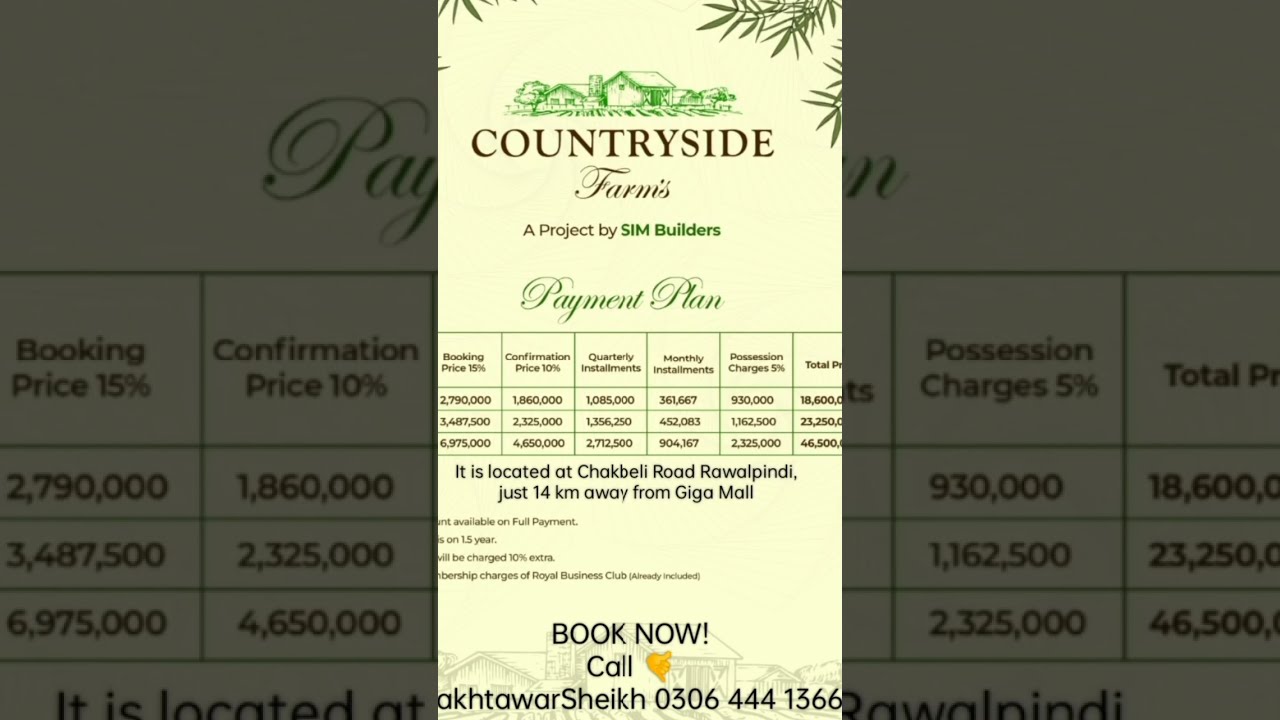This image depicts a detailed advertisement, possibly a screenshot or photograph, targeting potential clients for Countryside Farms. The ad is structured within a pamphlet approximately the size of a smartphone screen. Featured prominently at the top, against a yellow backdrop, is a green illustration of a farmhouse surrounded by a field with green leaves peeking in from the upper corners. Beneath the image, the text "Countryside Farms" is highlighted, with "Countryside" in brown block letters and "Farms" in an elegant brown italicized script.

Following the title, the ad mentions that this is "a project by Sim Builders," presented in standard green font. Detailed below this heading is an organized payment plan: "Booking Price - 15%" and "Confirmation Price - 17%" are both noted, alongside quarterly installments. Each detail is carefully laid out in a chart format with three distinct columns.

The bottom section of the ad includes practical information about the location and contact details. It states that Countryside Farms is situated at Chack Valley Road, Rawalpindi, approximately 14 kilometers from Giga Mall. Lastly, a clear call to action invites prospects to "book now," providing a contact phone number: 0306-444-1366. The polished presentation of the ad's information makes it easily digestible for viewers, ensuring clarity and engagement.